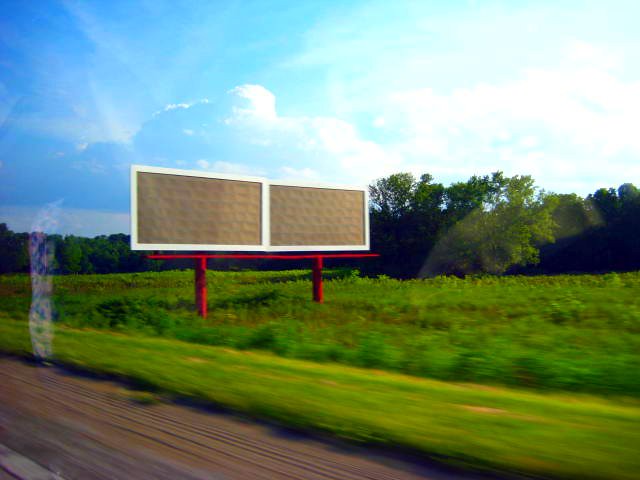This daytime outdoor photograph, taken from a moving car, captures a countryside scene featuring a blue sky that transitions from an incredibly light blue at the top to a medium blue further down. The sky has a few clouds that are faint and blend into the background. Below the sky, the horizon is marked by a tree line that spans from left to right, with more defined trees to the right and some further back to the left. 

A key element in the photograph is a set of two rectangular roadside billboards mounted on two reddish poles. These billboards, positioned just left of center, are blank, displaying only tan surfaces with white borders that give them a corkboard-like appearance. The billboards, sitting atop a red platform, are viewed from a slight three-quarter angle, creating shadows that fall to the left due to sunlight coming from the upper right. 

The image also shows the foreground details in slight blur, including an overgrown field to the right and the edge of a road with some dirt on the shoulder to the left. The blurring indicates the motion of the car from which the photo was taken. Additionally, there is a faint reflection in the car window, possibly of someone's clothing, adding to the sense of motion.

This serene image melds together the elements of nature, man-made structures, and a fleeting moment captured through the lens of a moving vehicle.